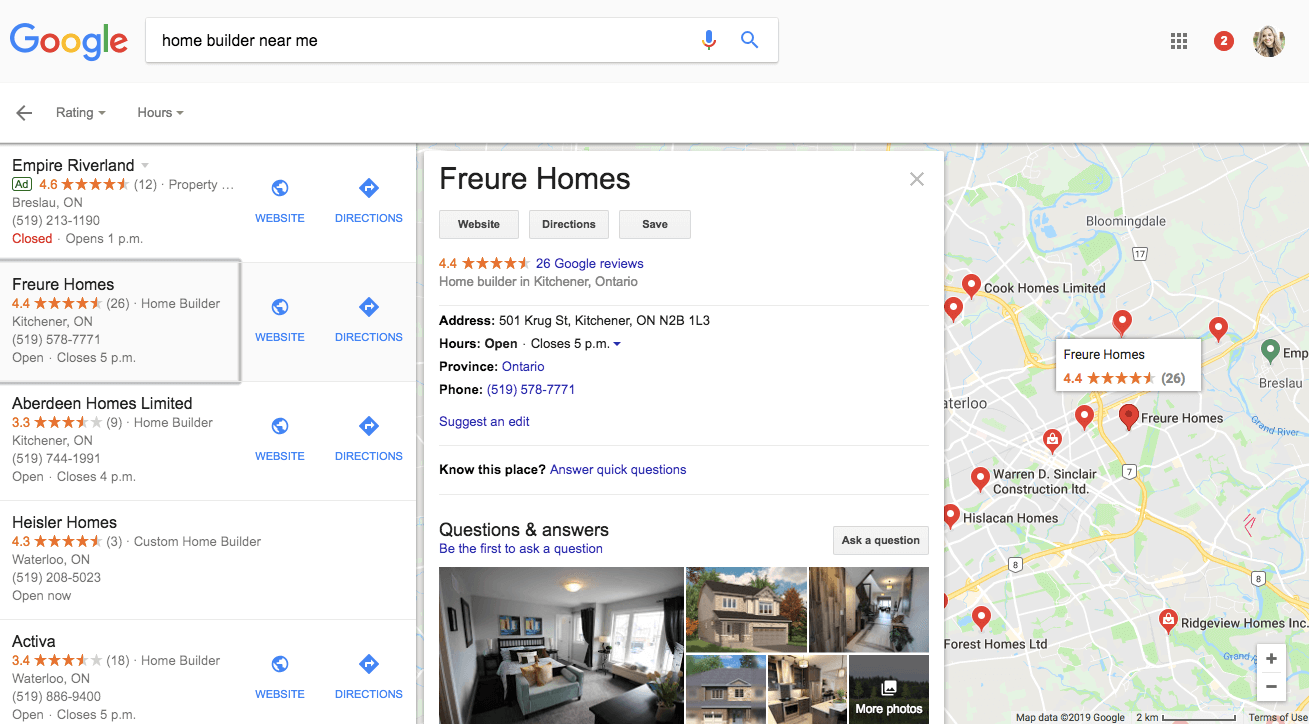This is a screenshot captured in landscape mode. The background is primarily gray, extending from the upper left corner to the upper right. In the upper right corner, there is an avatar of a young woman with long blonde hair. To the left of the avatar, there is a circle with the number "2" inside it. Further left, there is a grid icon consisting of nine squares arranged in three rows.

Towards the upper center of the screenshot, there is a Google search bar with the query "home builder near me" typed in. At the end of the search bar, there are two icons: a microphone and a search icon. To the left of the search bar, the Google logo is visible. Below the search bar, there are navigational elements including a back arrow, a rating with a down arrow, and "Hours" with a down arrow.

The main content is divided into three columns. The first column on the left lists five home builders:
1. Empire Riverland (not marked as an ad)
2. FR eure homes (highlighted with a gray background)
3. Aberdeen homes
4. Heisler homes
5. Activa

Each listing includes options for "Website" and "Directions".

The second column, which has a white background, focuses on FR eure homes. It features three buttons: "Website", "Directions", and "Save". FR eure homes has a rating of 4.4 out of 5 stars, marked in orange. Below the rating, there are links to 26 Google reviews, indicating it is a home builder located in Kitchener, Ontario. Their address, hours of operation, province (Ontario), and phone number are all clickable blue links. There is also an option to "Suggest an edit."

The third column reveals part of a Google Map displaying the location of FR eure homes, partially covered by the previous elements.